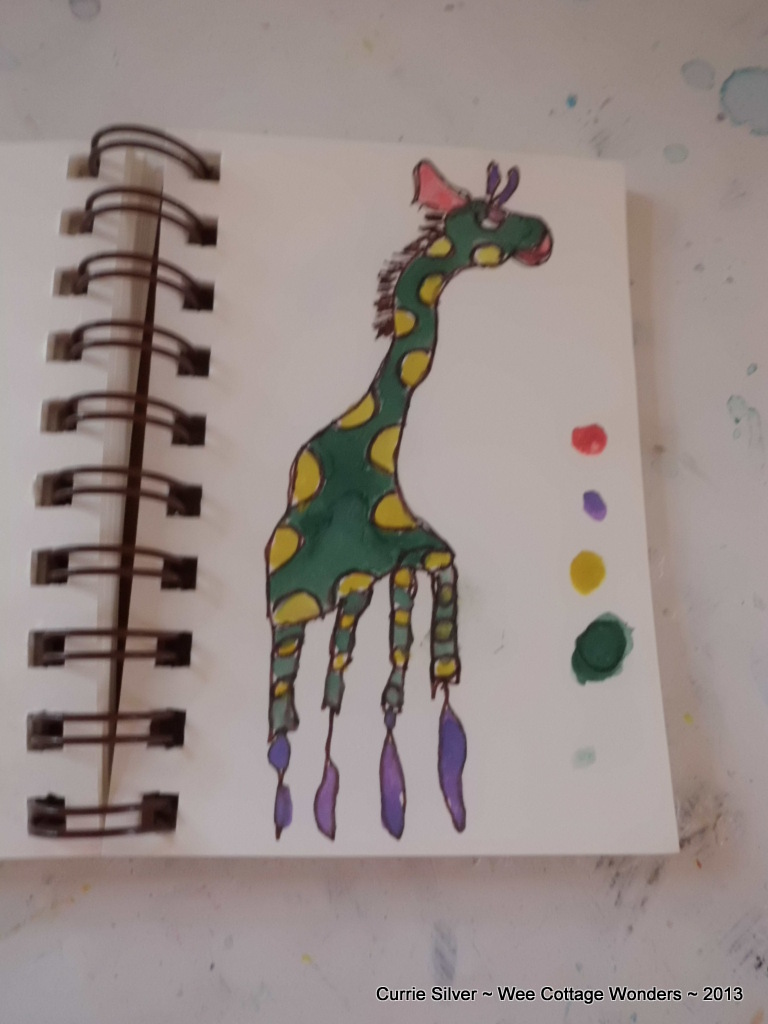This image captures a child's imaginative art project in a small, wire-bound sketchbook. The book is secured by approximately 15 wire rings along the left side, holding white, unlined pages designed for watercolor art. The focus of the sketch is a fantastical giraffe-like creature facing left, painted predominantly in dark green with lighter green and yellow polka dots. Its slender, elongated neck and head, adorned with two small horns, help maintain its giraffe-like appearance despite its unconventional coloring. The ears are a vivid pink, the mane is black, and the nose stands out in bright red. The legs of the creature are green down to the knees, then transition to bright purple, balloon-like shapes at the bottom, giving an impression of inflated, dangling bags or hooves. On the right side of the page, the young artist has tested a few colors, visible as four small, colored balls in green, yellow, blue, and red. At the bottom of the artwork, a watermark in black print reads, "Curry Silver, Wee Cottage Wonders, 2013," indicating either the artist's or photographer's signature. The backdrop of this photographed art is a white, slightly dirty table.